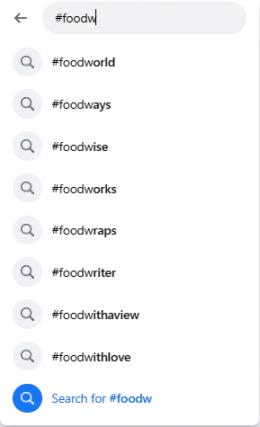The image depicts a search interface for different hashtags. At the top left corner, there is a dark grey arrow pointing to the left. Adjacent to the arrow is a long, rounded rectangle in light grey. Inside this rectangle, the text "#food w" appears in black, with a cursor indicating that the user is still typing.

Beneath this search bar are several suggested hashtags, each prefaced by a magnifying glass inside a grey circle. The first suggestion reads "#foodworld," followed by "#foodways," "#foodwise," "#foodworks," "#foodwraps," "#foodwriter," "#foodwithaview," and "#foodwithlove."

At the bottom of the list, there is a blue magnifying glass icon within a circle, featuring a white magnifying glass symbol inside. Next to this icon, the text "Search for #food w" appears in blue.

The entire interface is set against a white background. On the bottom and right edges of the image, a dark grey line marks the boundary where the screenshot is cut off from the rest of the image.